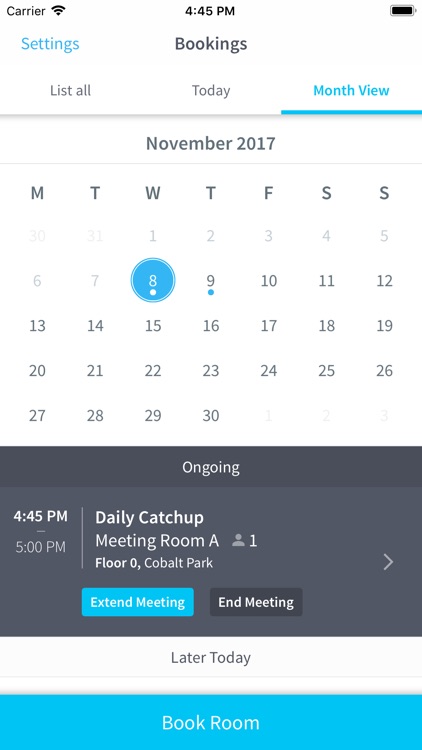The screenshot captures a smartphone's screen against a white background. In the top left corner, the screen displays the text "Carrier" and a black Wi-Fi symbol. The current time, "4:45 p.m.", is shown in black in the center, while the battery life indicator, which is completely full, is on the right.

Below "Carrier" is the blue "Settings" icon, and beneath the time, "Booking" is written in black. To the right of "Today", "Month View" is highlighted in blue with an underscore line below it. The text "November 2017" follows, with a gray horizontal line beneath it, and the letters representing the days of the week—Monday through Sunday—are listed horizontally. The calendar starts on Wednesday, the 1st, and ends on Tuesday, the 30th.

Beneath this section, a black box with white text reads "Ongoing" in the top center. On the left side within this box, it states "4:45 p.m. below that it says 5 p.m.". A vertical white line divides this information from the text on the right, which reads "Daily catch-up meeting, Room A", with a person icon and the number "1" next to it. Below "Meeting Room," it indicates "40 Colbert Park".

Further below are two buttons: "Extend Meeting" on the left in blue, and "End Meeting" on the right in black. Below this, on a white background, it says "Later Today". At the bottom of the screen, there is a blue button labeled "Book Room".